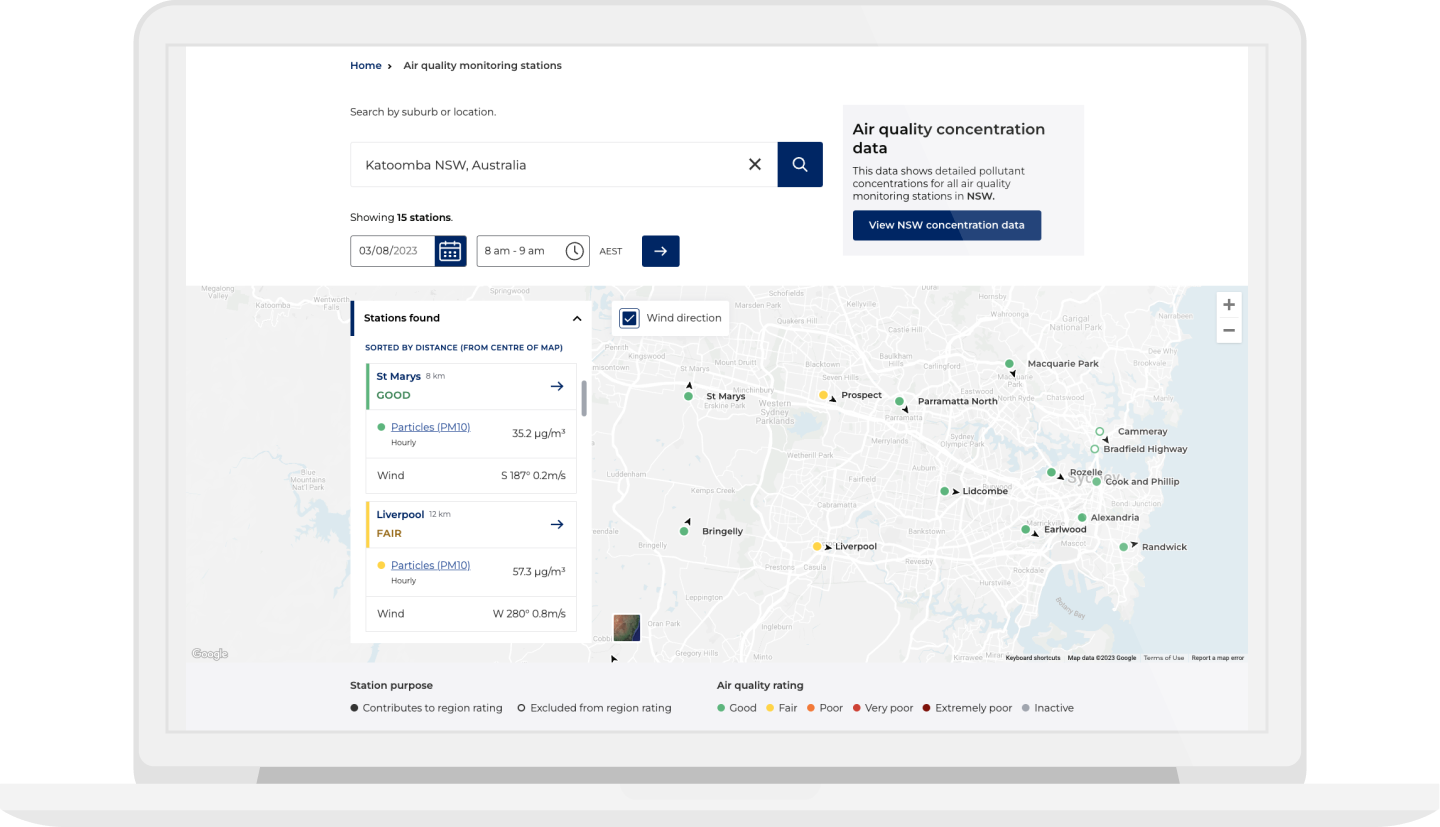A detailed map of Australia is displayed, with a highlighted section showcasing the town of Katoomba, NSW, Australia. The word "Home" is written in blue at the top, with a black arrow pointing towards air quality monitoring stations. Below Katoomba, the map indicates 15 air quality monitoring stations in bold black letters. 

At the bottom of this section, a date is provided: 03/08/2023, presented on a white calendar icon against a dark blue background. Adjacent to the date, a time range is shown: 8 a.m. to 9 a.m., along with a clock icon. The time zone AEST is also specified, followed by a blue square with a white arrow pointing to the right.

In the top right-hand corner, a light gray rectangle contains bold black text: "Air Quality Concentration Data." Below this, additional text in black states, "This data shows detailed pollutant concentrations for all air quality monitoring stations in NSW," with NSW in bold black. A dark blue rectangle features white text instructing, "View NSW Concentration Data."

On the left-hand side, another white rectangle has the heading "Stations Found" in black text. Below this, in blue text, it says "Sorted by distance (from center of map)."

A table displays various air quality data:
1. St. Mary's - A rectangle with a dark green line features bold blue text "St. Mary's" and beneath it, in green, the word "Good." On the right, a dark blue arrow points to additional details. A green circle icon follows, indicating particles (PM 10) in hyperlinked blue text with "Hourly" beneath. The concentration reads 35.2 µg/m³. Below, wind data states S 187 degrees at 0.2 m/s.
   
2. Liverpool - A rectangle with a yellow line on the left shows "Liverpool" in dark blue text with "12 KM" in gray below, and "Fair" in brown. The right-hand side has a blue arrow. Another rectangle shows a yellow circle and "Particles (PM 10)" in blue text, with "Hourly" beneath. The concentration is 57.3 µg/m³. Wind data indicates West 280 degrees at 0.8 m/s.